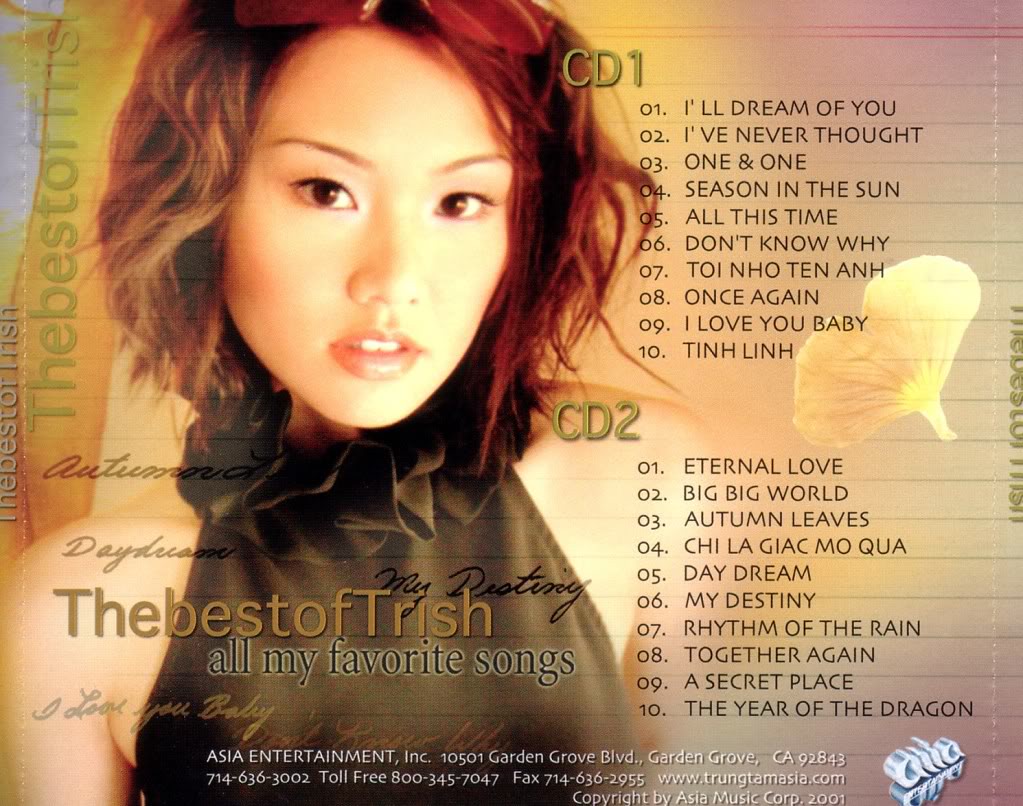The image depicts the back cover of a compact disc, showcasing album artwork titled "The Best of Trish: All My Favorite Songs." Dominating the left half of the cover is a large, detailed graphic of an Asian woman in her early to mid-20s, characterized by her short reddish or dark brown hair and soft features. Her expression is neutral, with her mouth slightly open, and she is wearing a sleeveless dark brown or black halter top with ruffles around the collar. 

The album's title, "The Best of Trish," is prominently displayed below her image in scrunched-up, brown font, almost appearing as a single word, followed by "All My Favorite Songs" in a bold, shadowed, all-lowercase script. Along the right side of the cover, two track listings are provided: one for "CD 1" and another for "CD 2," each containing ten tracks labeled 01 to 10. The first song on CD 1 is titled "I'll Dream of You," and the last track on CD 2 is "The Year of the Dragon."

The background of the cover features a complex design with pink and yellow hues, incorporating elements like yellow flower petals near the track listing and faint lines that give the impression of notebook paper. Alongside the left side, a vertical text reading "The Best of Trish" runs upwards, rotated 270 degrees. Cursive words and decorative elements are scattered across the background, adding to the intricate design.

At the bottom of the cover, the album provides information about the production company, Asia Entertainment Inc., including its address at 10501 Garden Grove Boulevard, Garden Grove, California, as well as multiple contact numbers and a fax number. The company's logo, "Asia," appears in a stylized white 3D font in the bottom right corner.